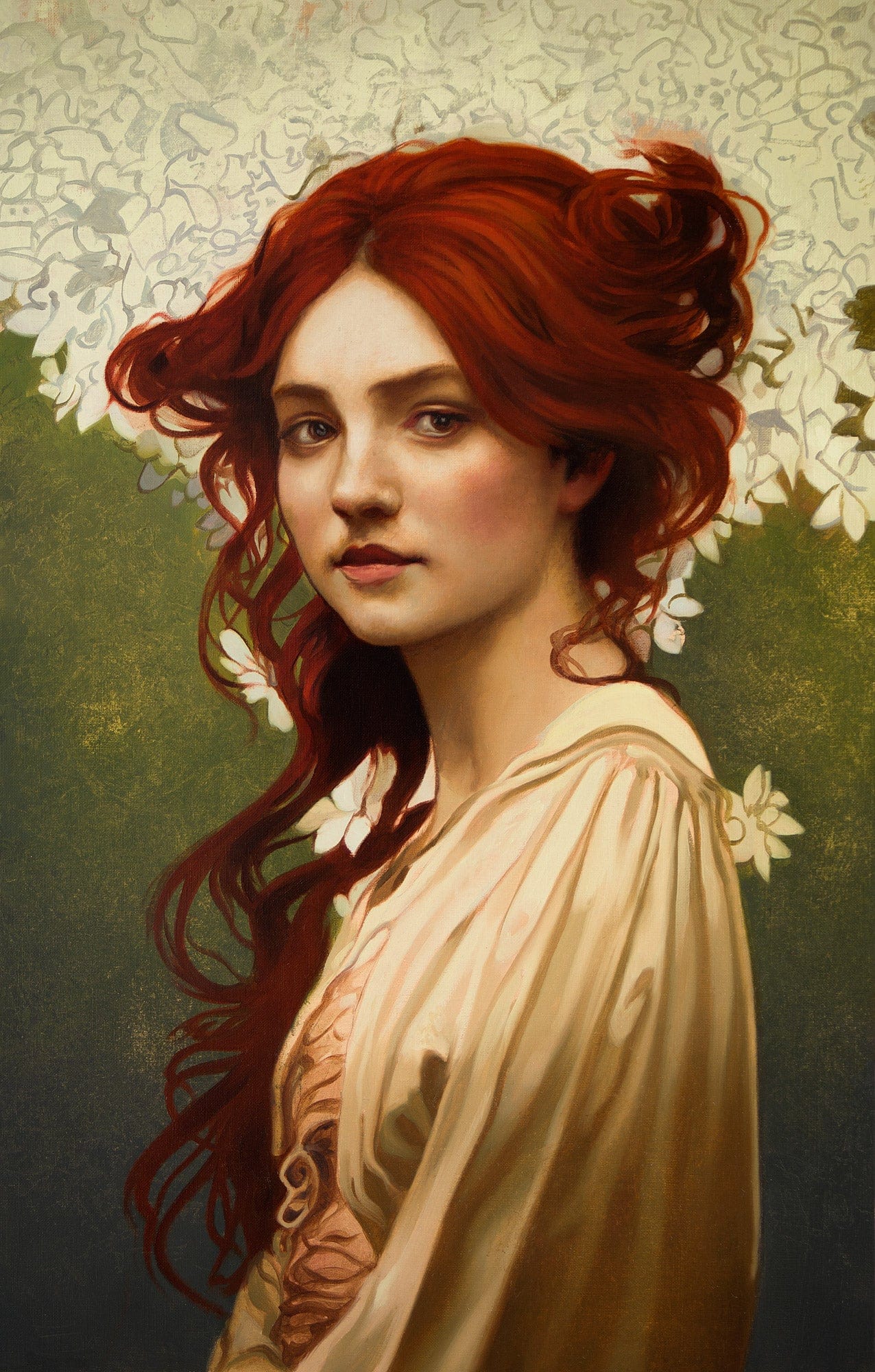The painting features a young girl with bright red, swishy hair that cascades down to her waist on the far side, while the front strands curl up around her ears. Her body is turned to the left, but her head is turned back towards the right, creating a sense of movement. She has fair white skin, dark brown eyes, and a slight pink hue on her cheekbones and lips, with a subtle shadow beneath her nose. She is adorned in a light cream-colored shawl draped over a pink blouse accented with gold stripes, the shawl displaying ripples down her shoulders. 

The background of the painting is intricate and dynamic. Above the girl’s head, there are detailed white drawings of flowers outlined in gray, covering the top third of the image. This floral design transitions into a mottled light green at the top, which gradually becomes darker towards the bottom, with specks of white interspersed throughout. The girl's red hair appears to defy gravity, swirling and whirling around her, adding an ethereal quality to the portrait.